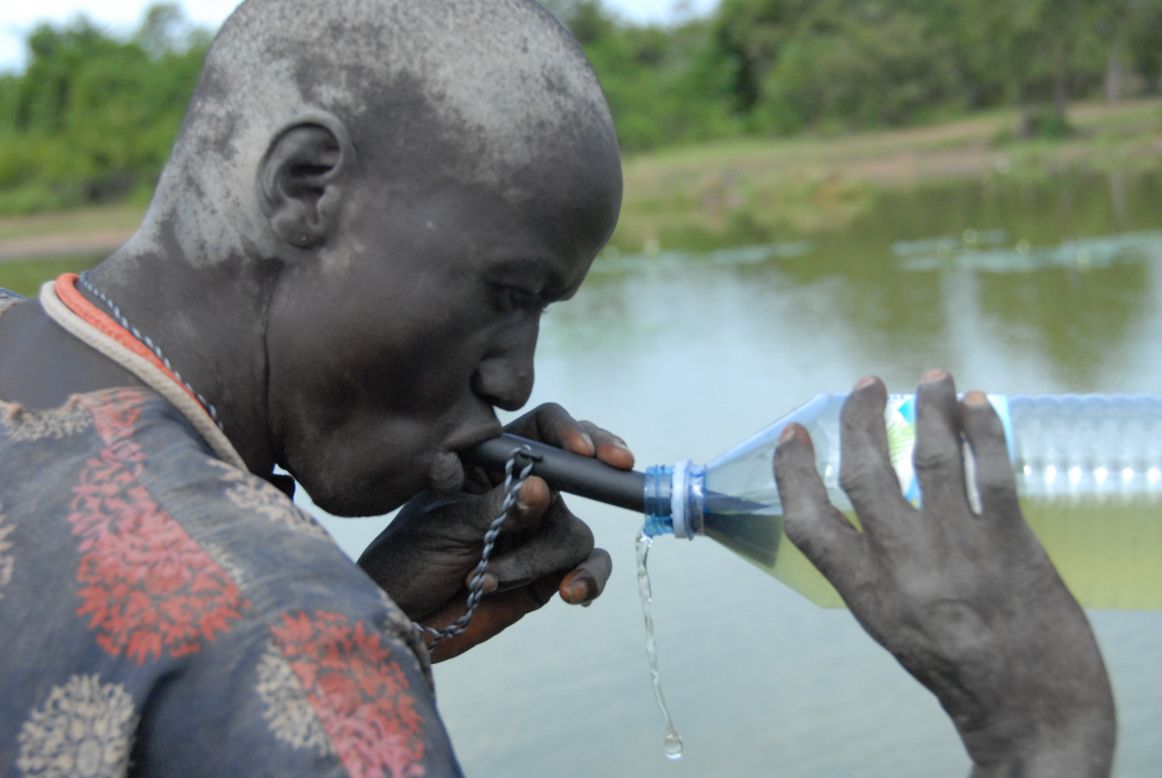In this close-up image, an elderly African American man, possibly African, is seen drinking water using a filter device. His complexion is very dark, and he has distinctive marks on his shaved head and neck, suggesting skin damage or a condition, giving parts of his head a white appearance. He is holding a clear plastic bottle filled with murky, yellowish-green water in his right hand. A thick black tube, which serves as the drinking filter, runs from the bottle to his mouth and is attached to a string around his neck. The man is wearing a shirt, which has been described as either brown, orange, and tan with a tree design or blue with red and white flowers. He is positioned with the background showing a slightly blurry lake that appears to have unclear, possibly algae-laden water. Beyond the lake, there is a shore lined with green grass and several trees, and the sky above suggests a nice day.